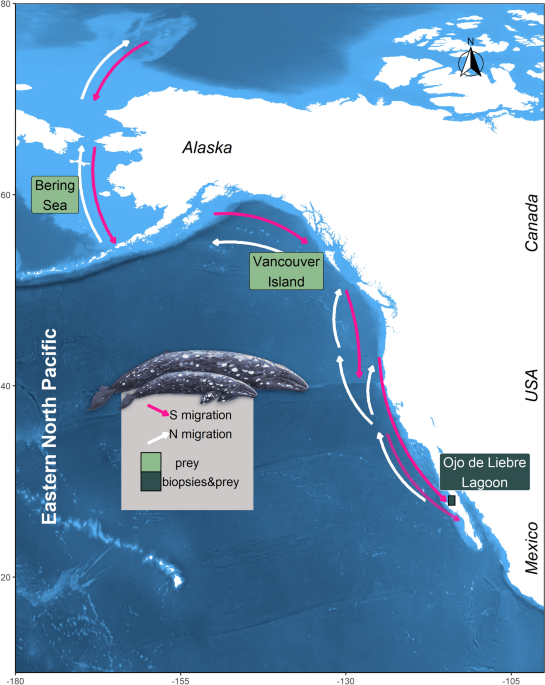This is a detailed illustration of the migration patterns of whales in the Eastern Northern Pacific. The map highlights the western portion of North America, including Alaska, Canada, the USA, and Mexico, with the northern Pacific Ocean shown in blue. Various arrows indicate migration routes: white arrows depict northward migration and pink arrows signify southward migration. There are notable labels such as the Bering Sea, Vancouver Island, and Ojo de Liebre Lagoon, each marked with green and black symbols representing prey and biopsy locations. The key on the map explains the color coding of the arrows and symbols. Additionally, two whales are depicted above the main graphic, one larger than the other, characterized by their black bodies with white spots. The map's layout includes a vertical list of countries along the right edge and a label "Eastern Northern Pacific" on the left side.